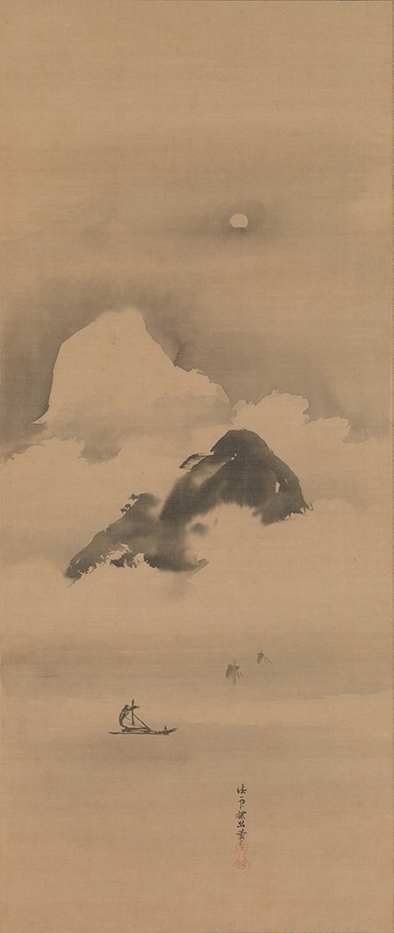This artwork is a minimalist Chinese painting on a vertical scroll with a tannish cream background. Crafted with light brush strokes, possibly using calligraphy or watercolor, it depicts a serene mountain in the distance enveloped by white clouds, rendered through the absence of color. Below the mountain, there is a faint portrayal of a body of water with a small black ship in the distance, slightly left of the center. The rest of the scroll features very light brown shading with moments of charcoal smearing to create abstract forms, enhancing the ethereal quality of the painting. Vertically aligned on the right side are Chinese characters, and at the bottom, a red seal, most likely the artist's signature. The composition presents a harmonious blend of subtle tones and minimalist elements, evoking a tranquil and contemplative atmosphere.